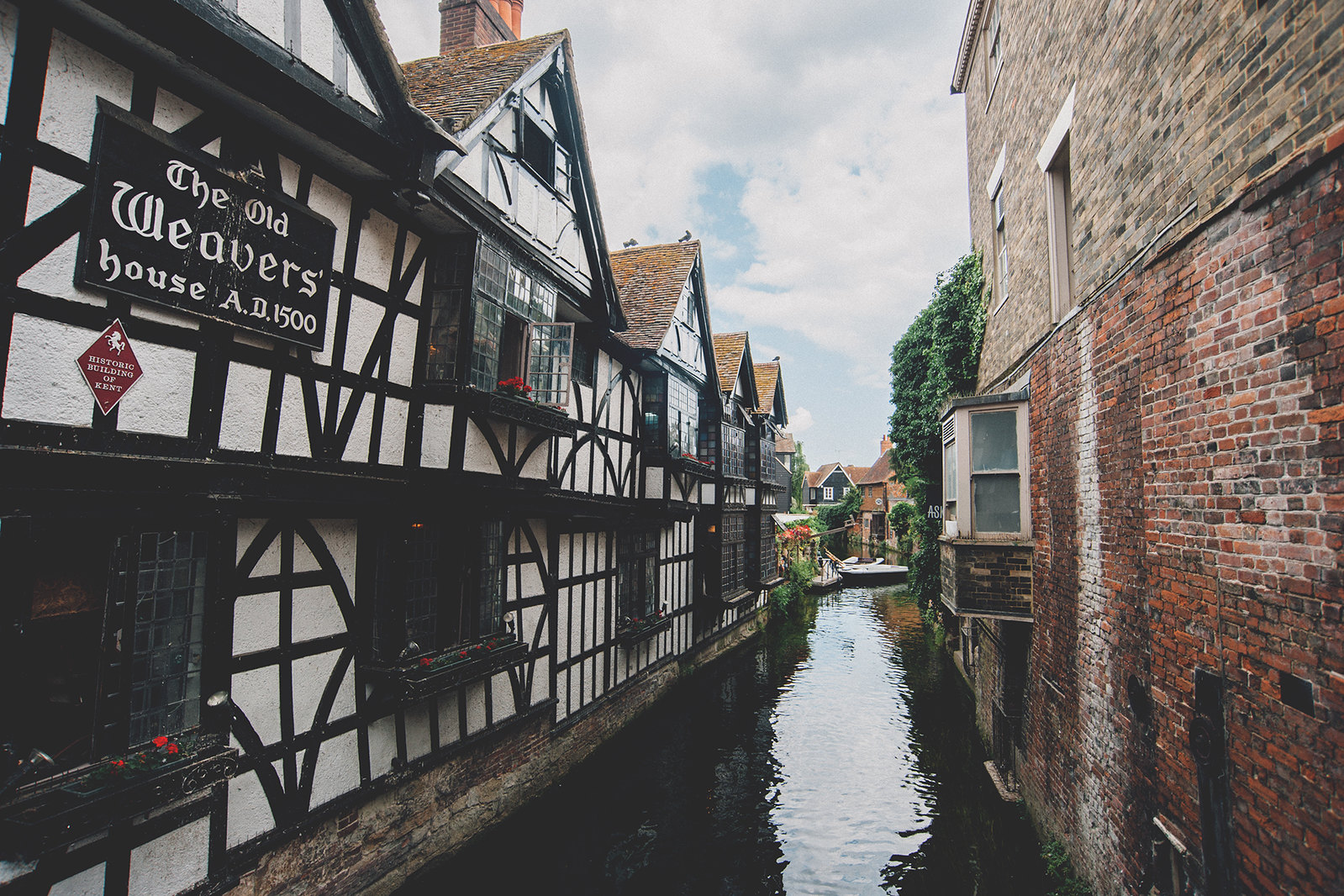This full-color daytime photograph captures an outdoor scene featuring a canal that runs between two distinct buildings. On the right side stands a large, old brick building with visible water damage and stains. It features a notable bay window and is located adjacent to a tree. To the left side, there is a striking German-style building that is primarily white with brown designs integrated into its structure. This building has numerous pointed roofs and windows, and bears a sign that reads, "The Old Weaver's House, A.D. 1500," which is rectangular and black with a triangular sign beneath it. The canal's dark water divides these buildings, suggesting either a river or a flooded street. The scene is complemented by a blue sky with several clouds overhead, indicating it isn't a particularly sunny day. Additionally, flowers are visible near the bottom left corner of the photo, further adding to the details of this picturesque setting.